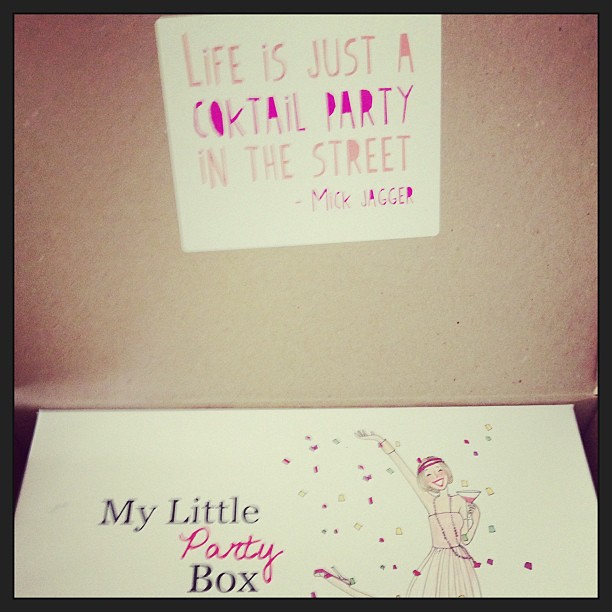The image depicts a whimsical scene centered around a white sticker with pink text that reads, "Life is just a cocktail party in the street," attributed to Mick Jagger. The background resembles a brown cardboard texture. Below the quote, there is another smaller white rectangular sticker with the text "my little party box" in a mix of pink and black fonts. To the right of this sticker is a lively cartoon illustration of a 1920s flapper girl, adorned in a pink dress, pink heels, and a pink bracelet. She has a playful and festive appearance, with a headband or beads around her forehead and a long beaded necklace. The stylish character is depicted with one hand holding a pink martini glass and the other arm raised high, possibly tossing colorful confetti, which surrounds her. Her pink lipstick, rosy cheeks, and jubilant expression further enhance the celebratory ambiance of the image.